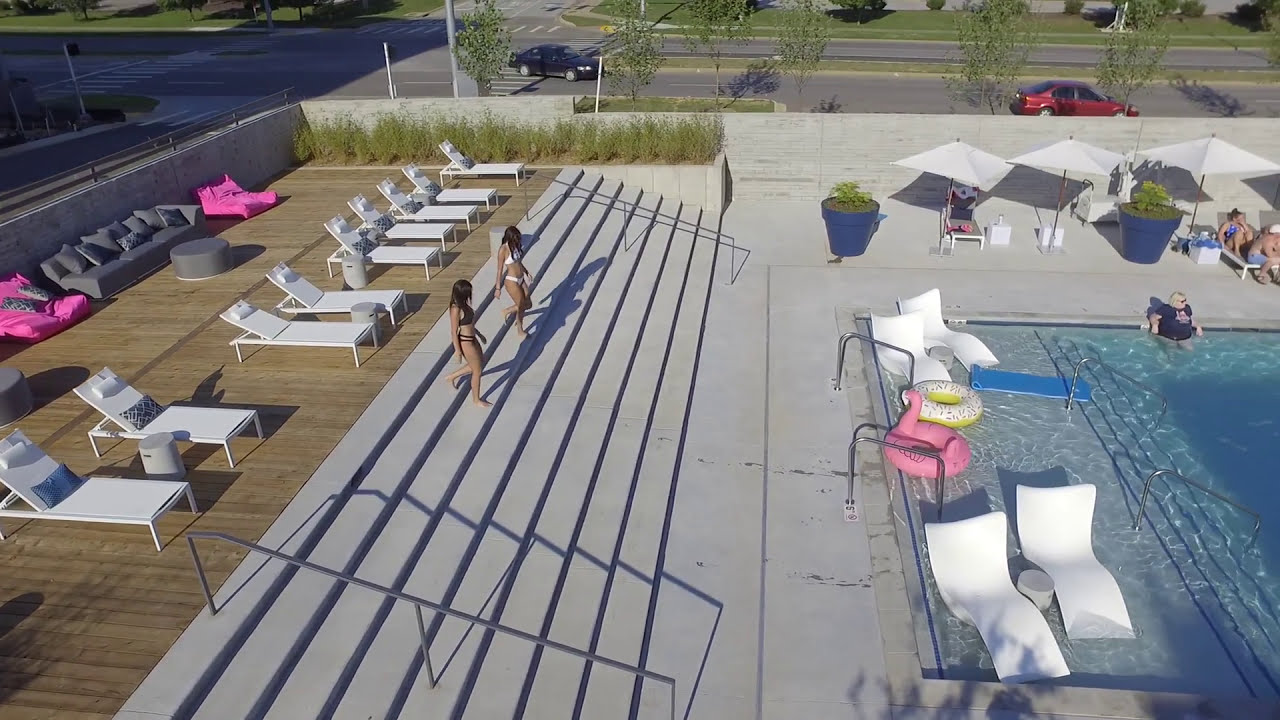In the foreground, two dark-haired women walk down concrete steps towards a pool, positioned on the right side of the image. Adjacent to them, in the top left corner of the image, stands a grey outdoor couch flanked by two pink chairs. A wooden deck is lined with a row of white lounge chairs. On the pool deck towards the middle right of the image, several white lounge chairs surround the pool area, complemented by a pink flamingo pool float. Three white umbrellas shelter lounging individuals in the top right corner. You can spot a street at the very top of the image, with two vehicles visible. The pool has a shallow end near which the women are heading, and various inflatable rafts, including white ones, clutter this end of the pool. Additionally, there is a larger woman standing in the pool, seemingly observing the descending women.